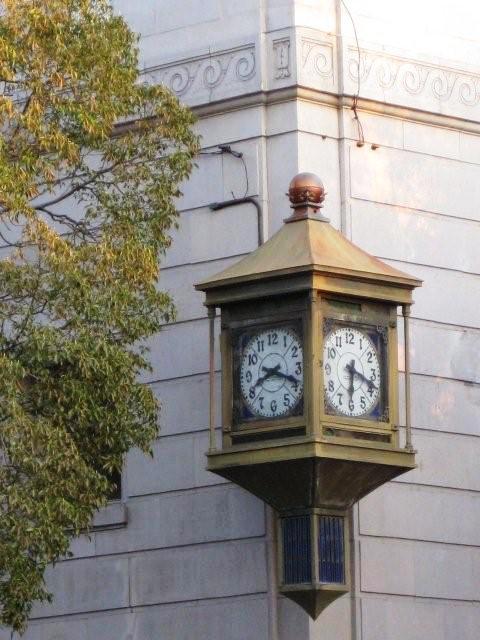This is a vibrant color photograph featuring a vintage clock situated at the corner of a historic building. On the left side of the frame, a partially visible tree showcases a gradient of leaves, transitioning from lush green at the bottom to a mix of green and yellow towards the top, indicating the changing seasons.

The building itself is richly adorned; its lower portion is constructed with sturdy grey bricks, offering a foundation of timeless sturdiness. Above the bricks, an intricately scrolled decorative plaster section captures the eye, exuding classic architectural charm. Just beneath this ornate plasterwork runs a horizontal line of golden brownish-beige, adding a touch of warmth and elegance to the facade.

The clock prominently stands out at the edge of the building, featuring two visible faces, and possibly more on the unseen side. It is encased in a luxurious gold container with a square rim, creating a striking frame around the clock itself. At the top of the clock's casing, the design converges towards the center, forming a canopy-like effect crowned by a spherical ornament, adding an element of grandeur.

The edge of the clock within the gold frame is a deep bluish hue, complementing the narrow rectangle of blue at the bottom of the clock's case. The clock face is pristine white, with distinctly black hands pointing to the time, which reads twenty minutes past six. The numerals from one to twelve are clearly marked, ensuring easy readability of this timeless piece.